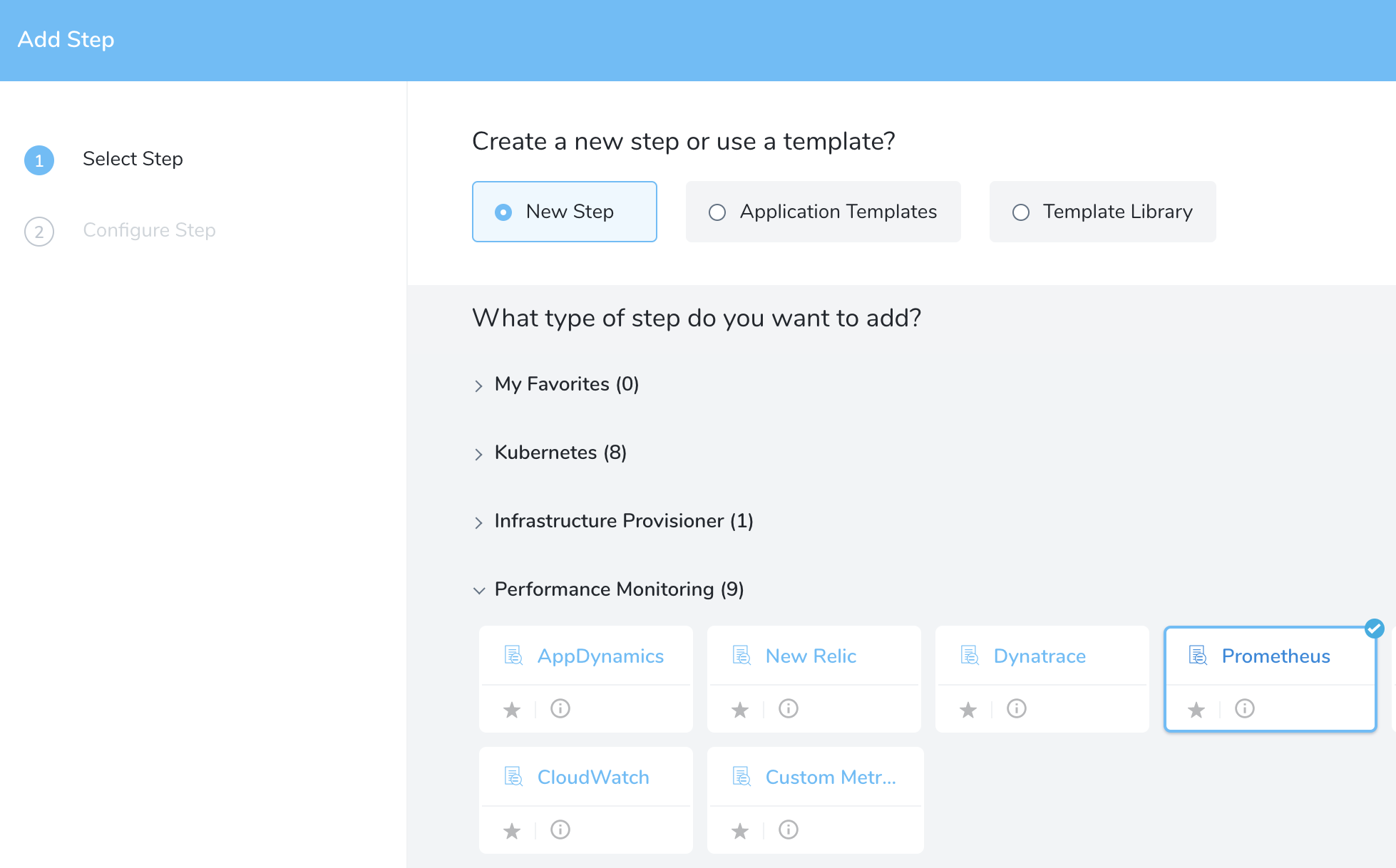This screenshot captures a desktop interface with a predominantly light color scheme that features a 50% white and 50% light gray background. The design includes a harmonious mix of black and blue text. A baby blue banner spans the top of the image, with the phrase "ADD STEP" displayed in white text in the upper left corner of the banner.

Beneath this banner, a white column on the left side contains two items: 
1. A blue circle with a white number "1" next to the faded text "SELECT STEP."
2. Below it, another circle with a faded number "2" followed by the text "CONFIGURE STEP." 

To the right of this column, the text "CREATE A NEW STEP OR USE A TEMPLATE" prompts the user with three clickable buttons: "New Step," "Application Templates," and "Template Library." The "New Step" button is highlighted in blue, indicating it has been selected.

Further down, the interface asks, "What type of step do you want to add?" Below this question, several options are presented. The user has chosen the "Prometheus" option, which is displayed in a blue text button box.

Overall, the interface is designed for adding and configuring steps, guiding the user through a process with clearly marked and interactive elements.